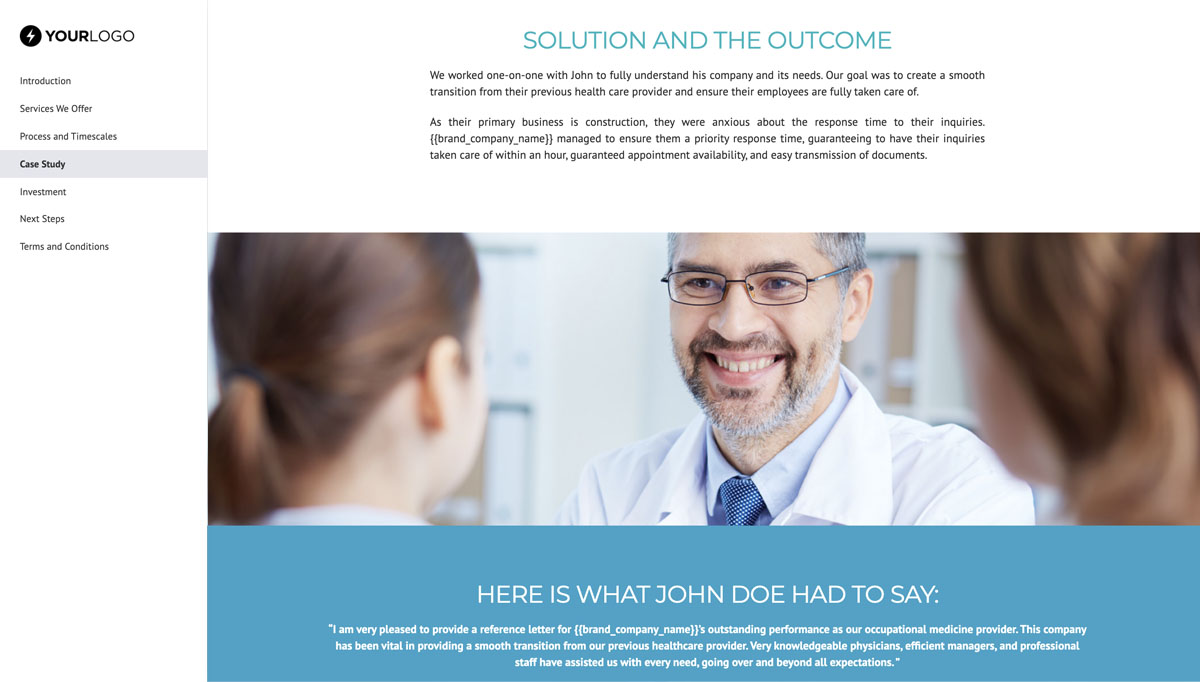This is a left-to-right horizontal image taken from a web page viewable on a computer or smartphone. The background is white, presumably the default color of the computer screen. 

On the left side, there's a black circle with a white lightning bolt symbol, indicating charging, beside the text "your logo." Below this section, there are clickable tabs labeled "Introduction," "Services We Offer," "Process and Time Scales," and "Case Studies," with the "Case Studies" tab highlighted in gray. Other tabs include "Investment," "Next Steps," and "Terms and Conditions."

Center-aligned on the page, written in light teal, uppercase letters, is the heading "SOLUTION AND OUTCOME." Below this, a detailed description states: "We worked one-on-one with John to fully understand his company and its needs. Our goal was to create a smooth transition from their previous healthcare provider and ensure their employees are fully taken care of. As their primary business is construction, they were anxious about the response time to their inquiries. Brand Name Company managed to assure them with a priority response time, guaranteeing that all inquiries would be addressed within an hour, along with guaranteed appointment availability and easy transmission of documents."

To the right, there is an image of a man wearing glasses and a white lab coat, smiling and conversing with two people. Below this image, the text reads: "Here's what John Doe had to say," followed by a testimonial expressing John's satisfaction with the performance.